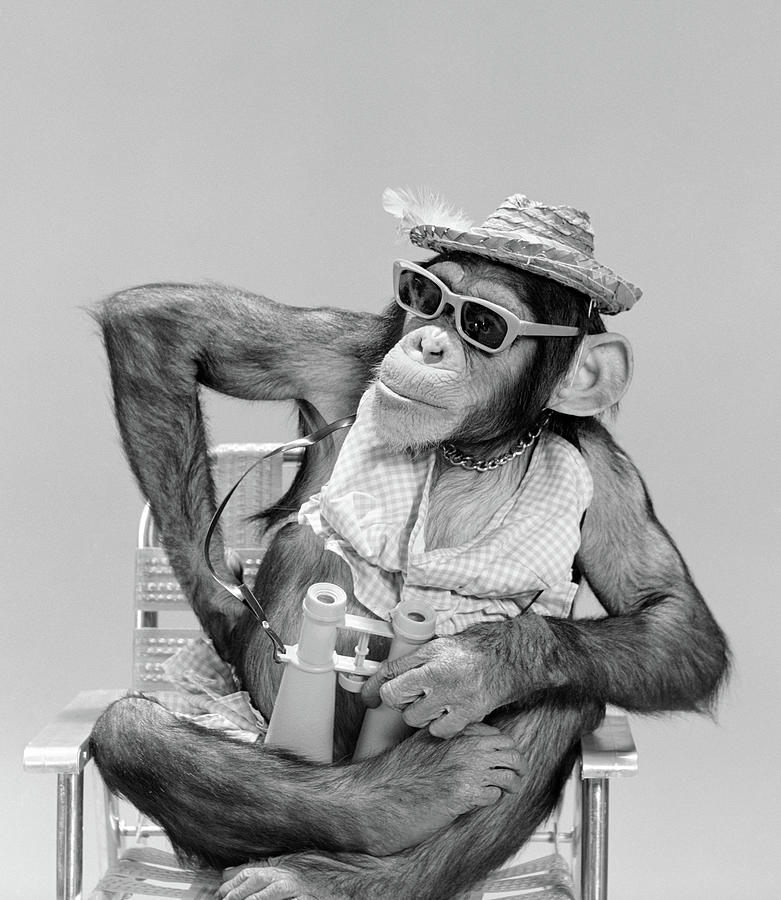This is a detailed black-and-white photograph featuring a chimpanzee dressed in an outfit that exudes quirky charm and a touch of sass. The background of the image is a simple, unadorned gray, which contrasts sharply with the vivid scene in the foreground. Seated cross-legged in a metal fold-out lawn chair, the chimpanzee is the center of attention. The primate sports a brimmed straw hat adorned with a feather, dark sunglasses, and a chain necklace. Draped over its torso is a tank top blouse that adds to its casual yet stylish appearance. 

Adding to the whimsical nature of the photo, the chimpanzee's right arm (on the left side of the frame) is cocked to a 90-degree angle, with its hand firmly on its hip, striking a confident and somewhat sassy pose. The left arm holds a pair of binoculars, which are slung around its neck by a strap, and the legs are folded comfortably in the chair. The chimpanzee's gaze is directed off to the right side of the image, giving the impression of it looking into the distance or surveying its surroundings. Overall, the composition combines elements of humor, style, and curiosity, capturing a moment of anthropomorphic whimsy.